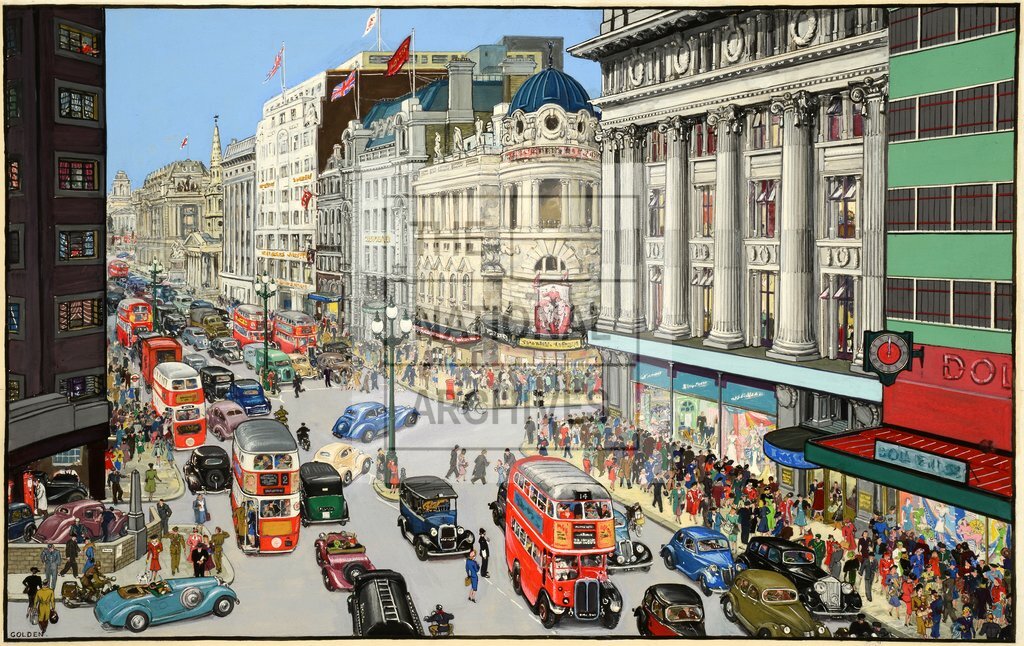This is a vibrant, detailed drawing depicting a bustling city street, likely from mid-20th century London, possibly around the 1950s. The scene is crowded with old-style cars and several iconic red double-decker buses, six of which can be seen traveling down the busy street. The sidewalks are teeming with people, some crossing the road, others gathered around the storefronts lining the right side of the street. The people are dressed in period outfits, with men in suits and hats and women in stylish skirts and dresses, indicative of the era. The architecture is characterized by tightly packed, tall Victorian buildings, approximately six to seven stories high, primarily gray and ornate in design. Notably, the closest building to the viewer on the right bears partially visible signage, "D.O. and possibly L.," and features a prominent clock showing 12 o'clock. Streetlights with three lamps each line the center of the street, painted green. Numerous flags adorn the buildings, including a clearly recognizable British flag and others with less distinct details. The blue sky overhead adds to the colorful and lively atmosphere of this chaotic yet captivating scene. A watermark reading "National Archives" stretches across the center of the image, and the bottom left corner bears the word "Golden."